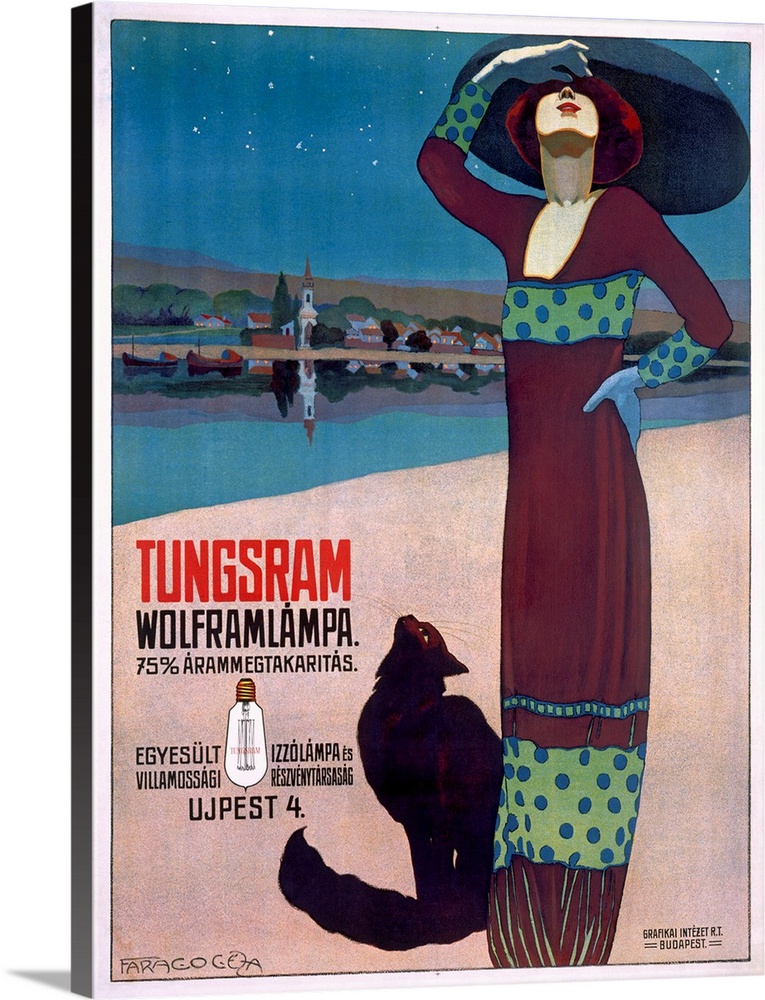This is a vertical Hungarian poster promoting Tungsram's Wolframlámpa, featuring the phrase "75% Aramegá Takharagatikás" on the left side. The bottom right corner of the poster credits Grafiákai Intezet R.T. Budapest. The central image depicts a tastefully dressed woman with red hair, adorned in a maroon dress detailed with green areas featuring blue polka dots and squares. She wears bluish-purple gloves and a large blue round hat, her right hand placed on her waist and her left hand shading her eyes as she gazes up at the sky. At her feet, a black cat mirrors her upward gaze. In the background, there is a townscape with a river, various buildings, and a notable church spire, all set against a blue sky with some greenery visible.